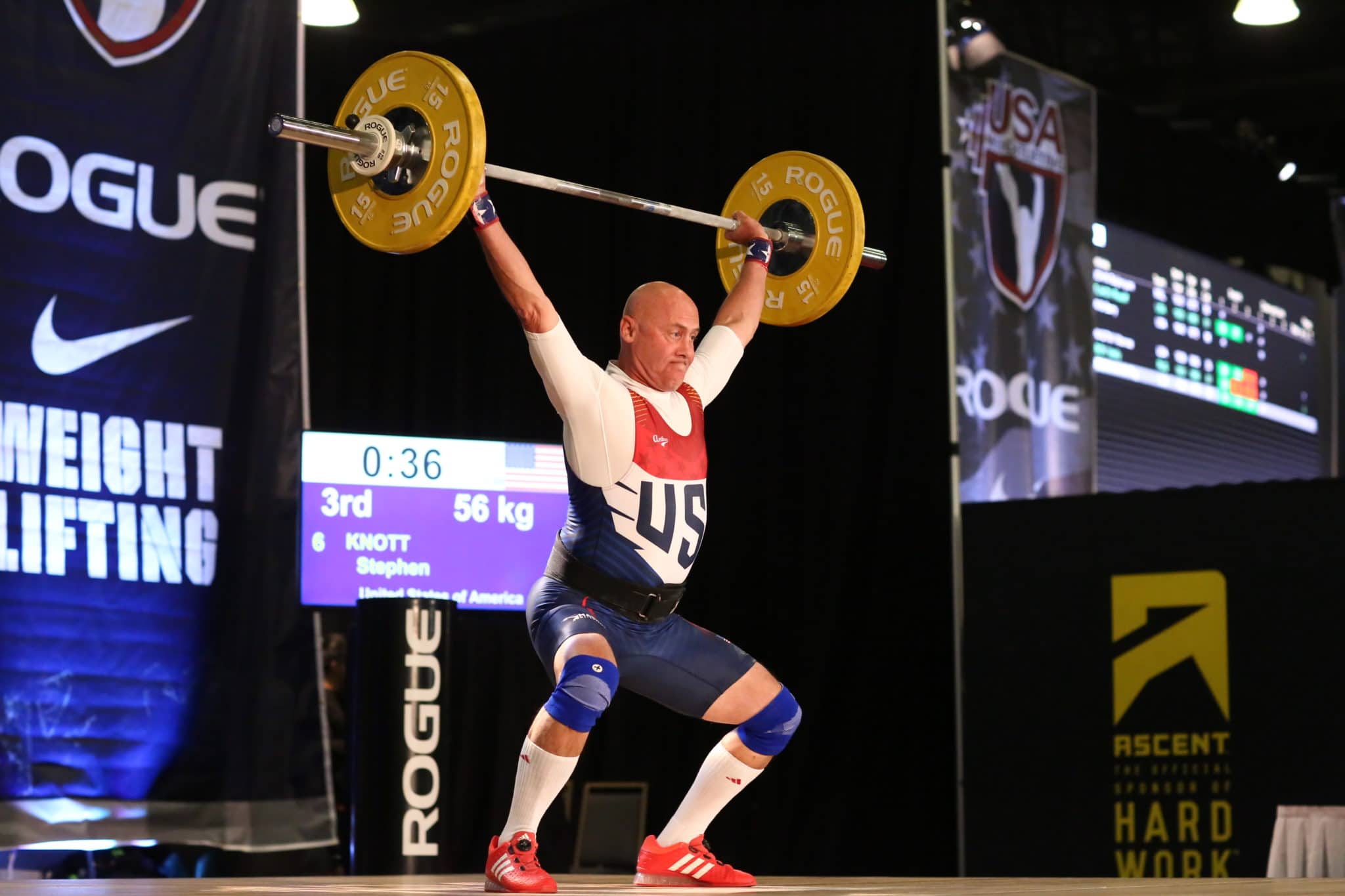In a vibrant, indoor weightlifting competition, the central figure—a powerlifter—is captured in mid-squat, holding an impressive barbell with large gold plates marked "Rogue" elevated overhead. The man, bald-headed and deep in concentration, showcases his strength while donning a white, elbow-length shirt beneath a red, white, and blue USA jersey. His attire is completed with dark blue shorts, blue knee pads, white socks, and striking red shoes featuring three white stripes. 

His stance is resolute against a backdrop filled with weightlifting paraphernalia and advertisements. To his left, a vertical sign also branded "Rogue" stands prominently. Above it, a TV screen on a purple background displays his standing—third place—with a timer counting down from 36 seconds and noting a 56-kilogram lift. In the far left of the image, a large banner showcases the words "Rogue" and a Nike logo followed by "weightlifting" in white letters. On the bottom right, a black banner highlighted with yellow text reads "Ascent Hard Work," emphasizing the dedication required in the sport. The detailed composition of the photograph vividly encapsulates the competitive spirit and intense focus required in the world of professional weightlifting.